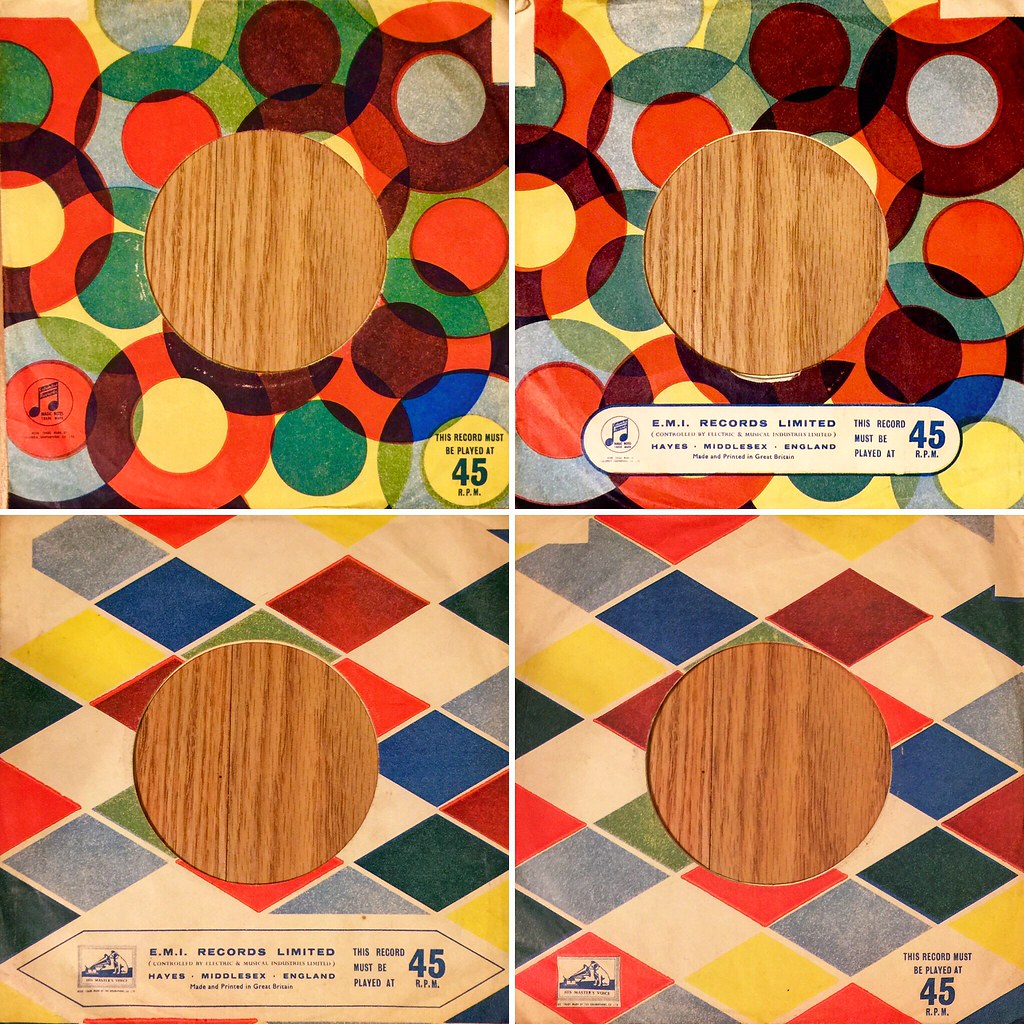The image features a detailed collage of four distinct sections, each showcasing identical wooden circular objects at their centers. Each section is marked by vibrant, recurring colors, including red, blue, green, yellow, and white, in various shapes such as circles and squares. In the top two sections, circular plastic elements in yellow, green, and red surround the central wooden piece. Both sections prominently display the text "This record must be played at 45 RPM" on the lower right corner, although the musical note symbol and text details differ, both incorporating "EMI Records Limited."

The bottom two sections mirror the top, maintaining the central wooden circular object theme. Both contain arrays of colorful diamond and square shapes and are similarly labeled with "EMI Records Limited" and "This record must be played at 45 RPM." Notably, the left bottom section includes additional imagery like the RCA logo featuring a dog looking into a record player. The entire collage is encapsulated within a square rectangular frame, unified by its consistent color palette and repetitive text elements that highlight the required 45 RPM playback speed for the depicted records.